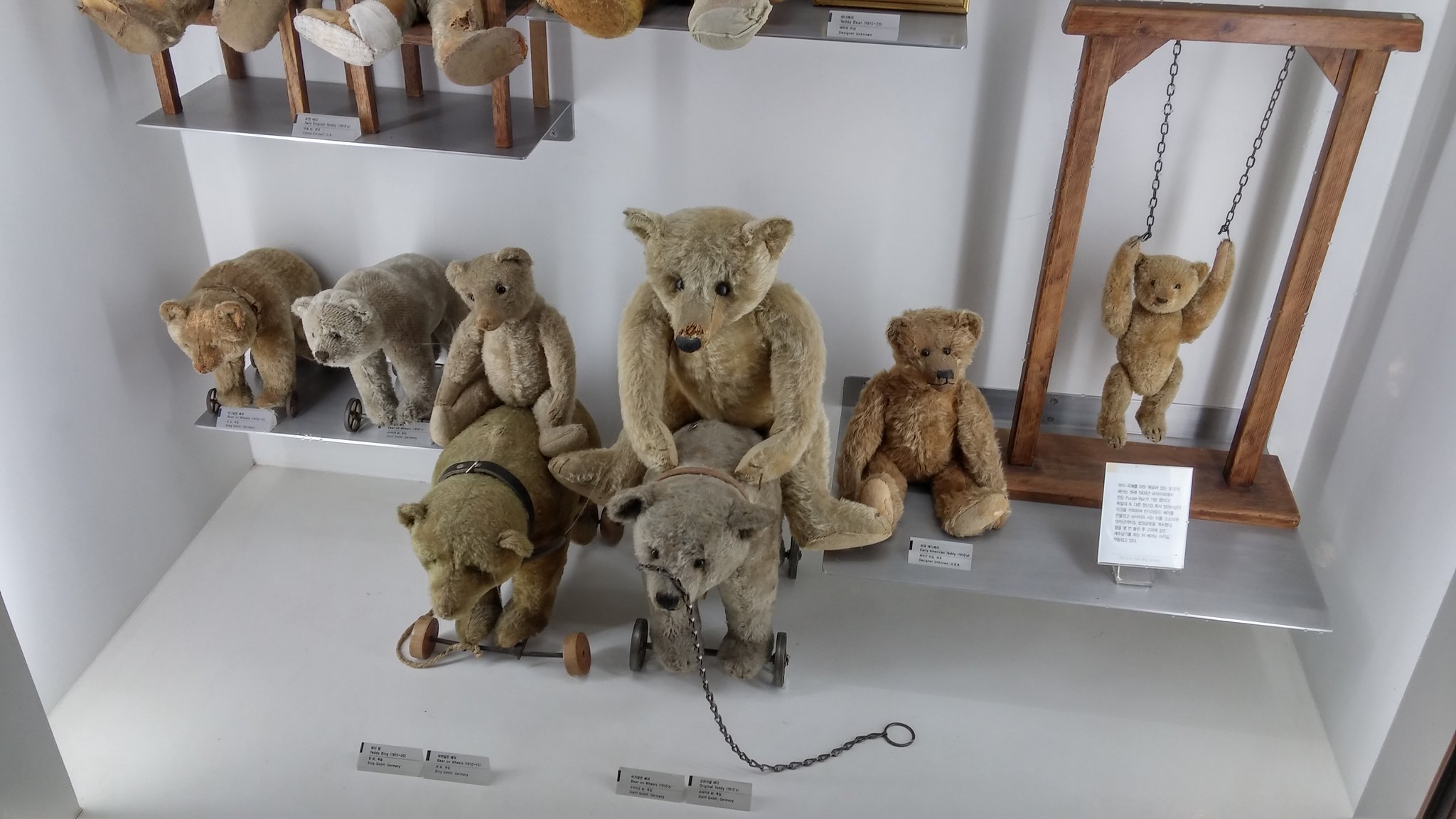The image depicts an intricate museum display featuring an array of meticulously crafted, high-end teddy bears. The teddy bears, all differing in shapes and sizes but uniformly jointed and meticulously stitched, appear to by made by the same esteemed manufacturer. At the top of the display, a small silver shelf holds three stools with teddy bear feet dangling over the edge. To the right, a brown scaffolding supports a swing or rings from which a small brown teddy bear dangles. Below this, three more teddy bears are showcased: one brown and one gray bear are positioned on all fours, with a smaller bear riding on the brown teddy bear, which has wheels attached to its feet. Similarly, another larger brown teddy bear on all fours, also with wheels, has a gray teddy bear sitting on its back, and is equipped with a chain for pulling, suggestive of a toy wagon. Adjacent to this setup, another small shelf holds a seated teddy bear, with its head slightly tilted, gazing outward. The attention to detail in these teddy bears, coupled with their carefully arranged positions, evoke a whimsical aesthetic, reminiscent of circus bears performing tricks. The entire assembly underscores the craftsmanship and artistry employed in their creation, presenting a charming and nostalgic exhibit.